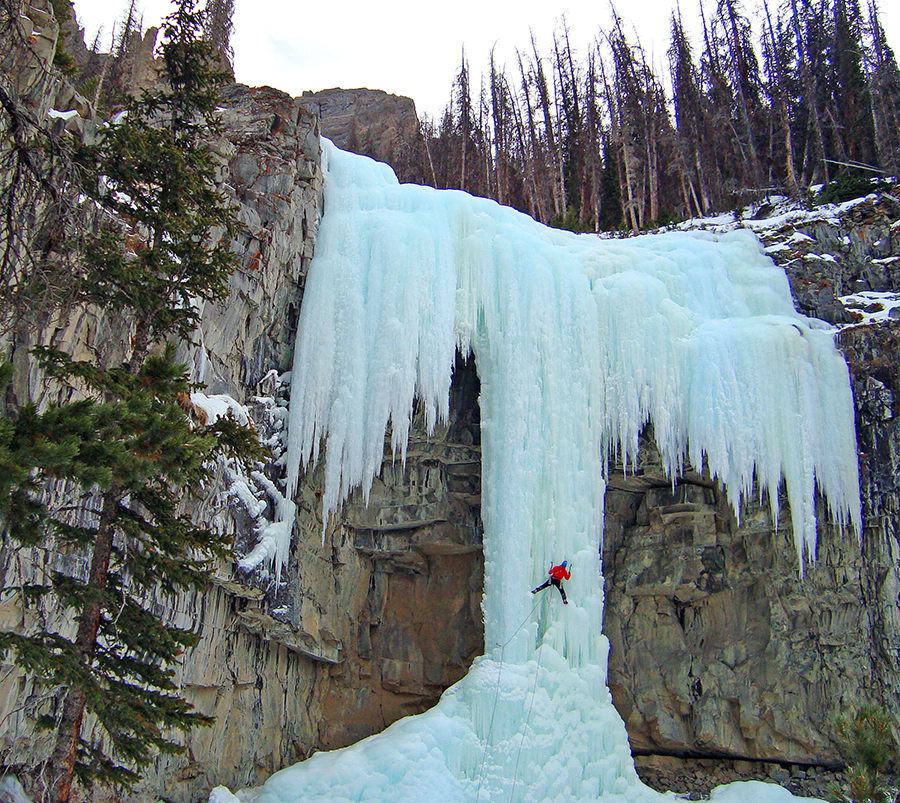The photograph showcases a striking frozen waterfall set against a majestic mountain backdrop in Cody, Wyoming, part of the Cody Ice Festival. This square-format, color image captures the sheer, rocky cliff face adorned with jagged white icicles cascading down from the top. At the center of this icy marvel, a climber is midway through their ascent. The climber, equipped with ropes and a harness, is wearing a distinctive orange jacket and black pants, facing away from the viewer. They are seen skillfully wielding ice picks, essential tools for navigating the frozen cascade. The image details a path of ice in the center, flanked by jagged icicles on either side. Tall pine trees are visible to the left and along the ridge at the upper right, adding to the natural splendor of the composition. This photograph is a testament to the exhilarating ice climbing opportunities and scenic beauty of Wyoming’s winter landscape.